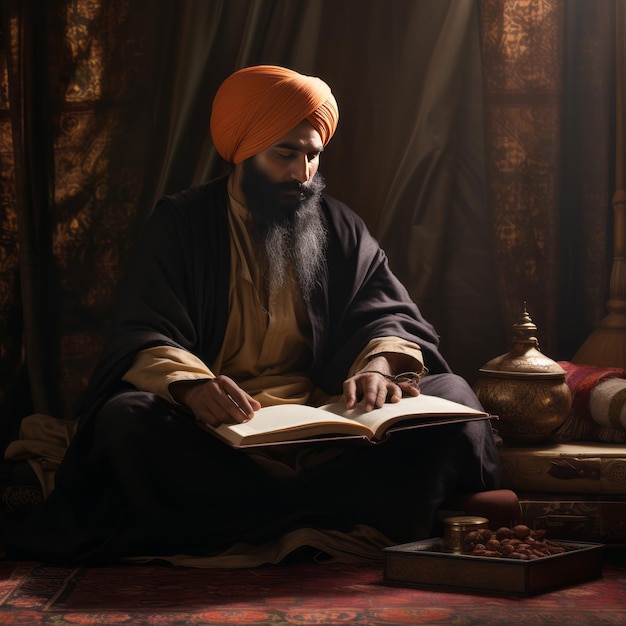The image depicts a man dressed in traditional Muslim attire, consisting of dark black and beige robes, with a distinctive bright orange turban wrapped around his head. He is sitting cross-legged on a carpeted floor, with a serious expression that suggests he is deep in thought or prayer. His long, spraggly beard transitions from a dark black at the base to gray and white at the tips, accompanied by prominent black eyebrows above his eyes, which seem closed or focused intently on the book in his lap. Both his hands are engaged with the book, his right hand poised to turn the page while his left index finger traces the line he is reading. Surrounding him are various objects, including a small gold container and a tray of grapes, suggesting a setting of contemplation or religious devotion. The background features ornate decorations and fabric-lined walls, with light illuminating the right side of his face.